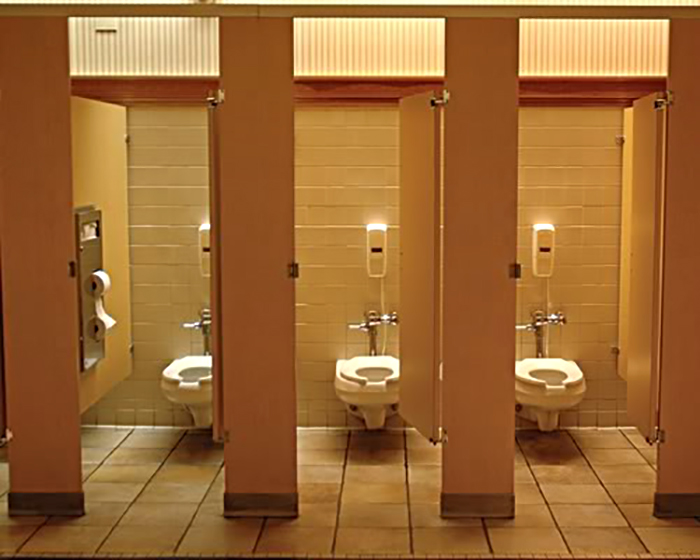The image captures a low-quality, yellowish-toned public bathroom with three open stalls. Each stall features a closed-seat white porcelain toilet, connected to silver flush pipes. Behind the toilets, white or yellowish containers, likely with a light on top, are mounted on light-colored, cinder block-type walls. Above this, there appears to be a striped wallpaper separated by a piece of wood trim. The floor is tiled in beige to yellowish-brown tones. The stall doors and partitions are a dark orange color. In the leftmost stall, a toilet paper dispenser holding two rolls is visible; the top roll has some paper unrolled and hanging down into the second roll.